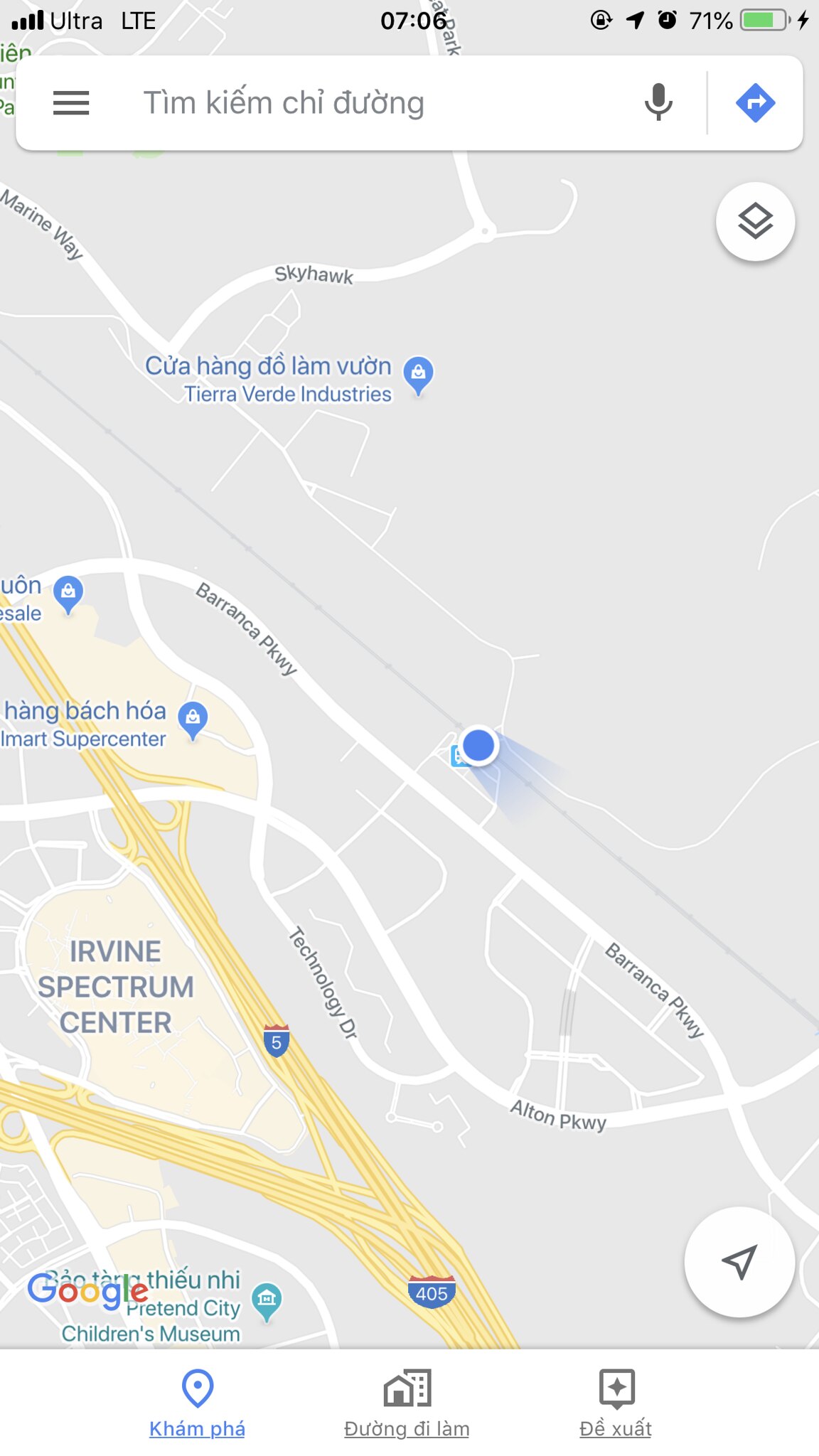A smartphone screenshot of Google Maps depicts a section of Vietnam with a notable gray area. This area is intersected by numerous white, winding roads and yellow highways marked with blue-red badges displaying their numbers. At the top of the smartphone screen, "Ultra LTE 706" is visible, indicating the device's network status.

In the search bar, text appears that resembles Vietnamese, reflecting the local language. At the bottom of the map, the familiar Google logo is present alongside the words "Irvine Spectrum Center."

Several English-named roads and landmarks are identified on the map, including Technology Drive, Alton Parkway, Marine Way, Skyhawk, and Tierra Verde Industries. The map also highlights Pretend City Children's Museum and Bronco Parkway. Additionally, a partially visible label reads "Super Center."